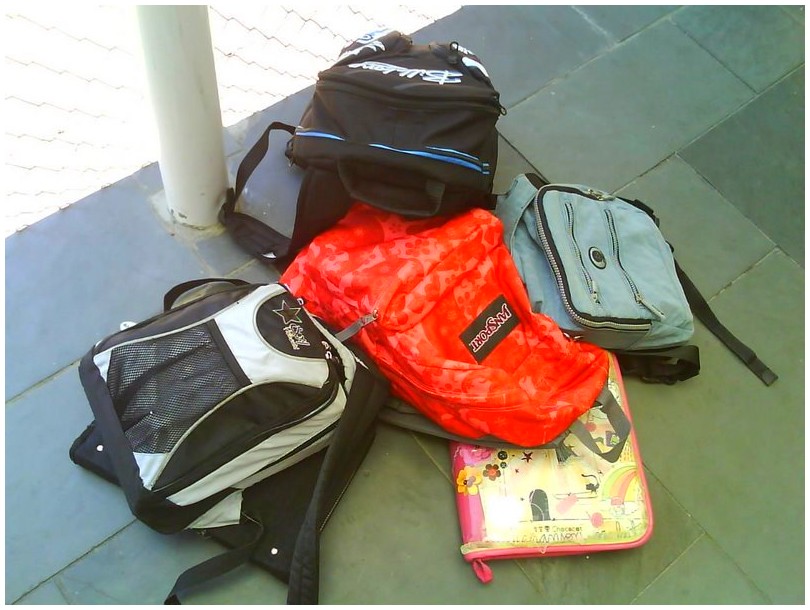In this outdoor photograph, set against a backdrop of green and gray stone tiles, a small pile of school backpacks is meticulously detailed. The focal point is the vibrant collection of bags laying next to a white pillar extending upwards towards the upper left of the frame, where bright sunlight or possibly a chain-link fence adds a contrasting brightness. Centered among the bags is a distinct Jansport backpack, displaying a red and peach colored pattern. Above this is a predominantly black backpack featuring white writing and blue stripes, identified as possibly from Billabong. To the left, a black and white backpack with a mesh pocket and a star can be seen, while to the right, there’s a smaller blue backpack. Completing the scene is a pink notebook featuring Disney characters and Chinese writing, further suggesting a school setting. The backpacks are arranged neatly, highlighting the varying colors and details against the stone tile flooring.